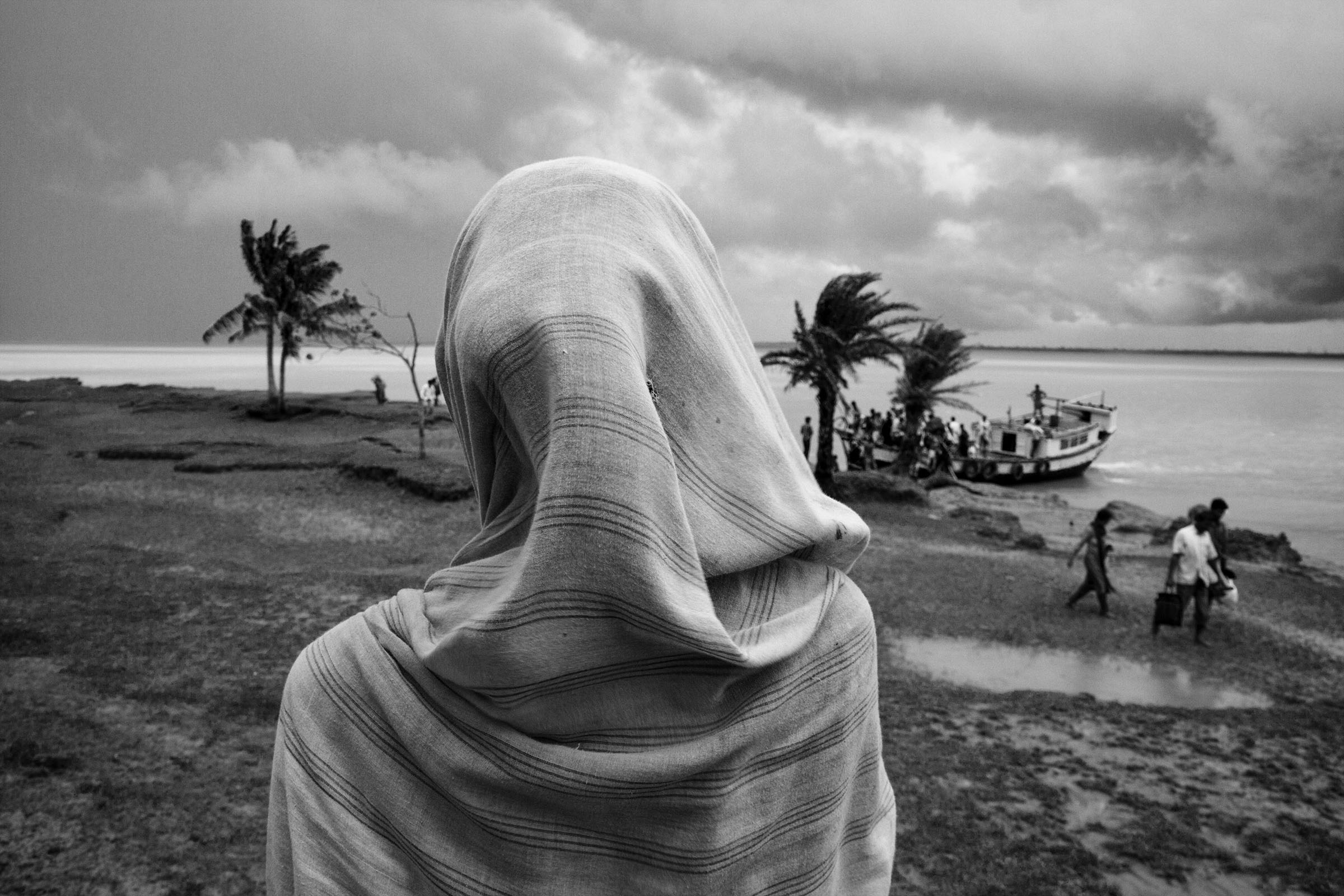This black-and-white photograph captures a dramatic, overcast sky filled with dark gray storm clouds. In the distance, a number of palm trees bend and twist dramatically in the gusting wind. On the right side of the image, the water blends almost seamlessly into the ominous sky above. Docked on the shore is a boat, with what looks like a large group of people either boarding or waiting to board. In the lower right corner of the image, three figures stroll along the muddy terrain, moving towards the right. Dominating the foreground, a figure stands with their back turned to the camera. Despite not revealing their face, the figure appears feminine and is cloaked in a layered and folded shawl that covers their head and shoulders. The stark landscape and the poised figure create a sense of solitude and contemplation against the impending storm.